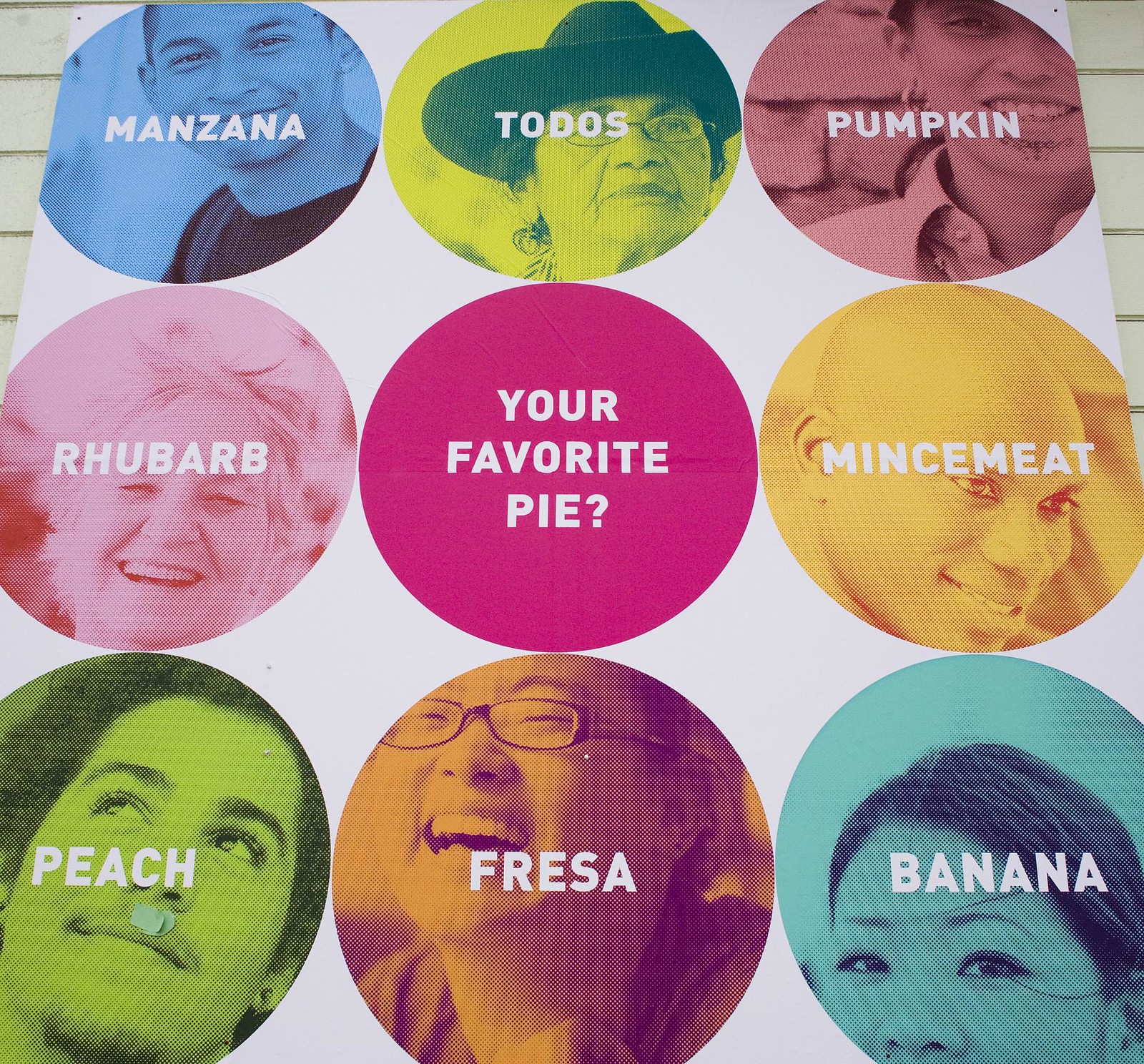The photograph shows a paper advertisement featuring a 3x3 grid of colorful circles, each containing a photograph of different people ranging from an older woman to a young boy. Each circle is a distinct color: blue, yellow, pink, green, orange, and has white text overlaying the images. The captions within the circles, starting from the top left and moving left to right, and then top to bottom, are: "Manzana," "Todos," "Pumpkin," "Rhubarb," followed by a magenta circle with the text "Your favorite pie?" and no photograph. Below that, the circles read "Mincemeat," "Peach," "Fresa," and "Banana." The advertisement is lying on what appears to be a table, possibly against a whiteboard with wooden slats visible at the corners, indicating a question asking readers about their favorite type of pie.